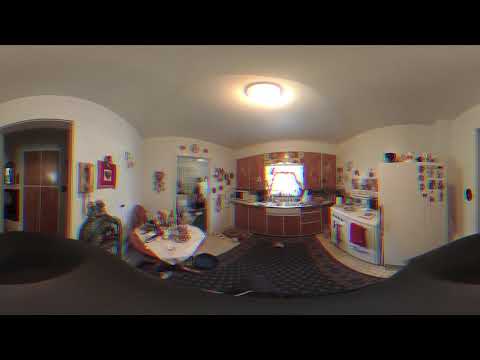This extremely blurry, horizontally rectangular full-color image, resembling the effect of viewing a 3D image without glasses or through a 360-degree camera, captures an indoor kitchen and dining area framed by a black border at the top and bottom. Despite the heavy distortion and blurriness, certain features stand out clearly. The kitchen on the right boasts a white stove and oven next to a similarly colored refrigerator, set against wooden cabinets and black countertops. Above the sink, centrally situated, a window lets daylight spill in, complemented by an overhead yellow light. To the left, the dining area features a round table covered with a white tablecloth, surrounded by chairs, while a nearby pantry with floor-to-ceiling cabinets adds to the kitchen’s storage. The room feels cluttered, with various items scattered on the table and atop the refrigerator. A hallway on the left leads to another door, and the dark-tiled floor is accented by a dark gray Persian rug. Overall, it presents a complicated blend of familiar kitchen elements distorted by unconventional photographic effects, with an apparent mix of daylight and artificial light.